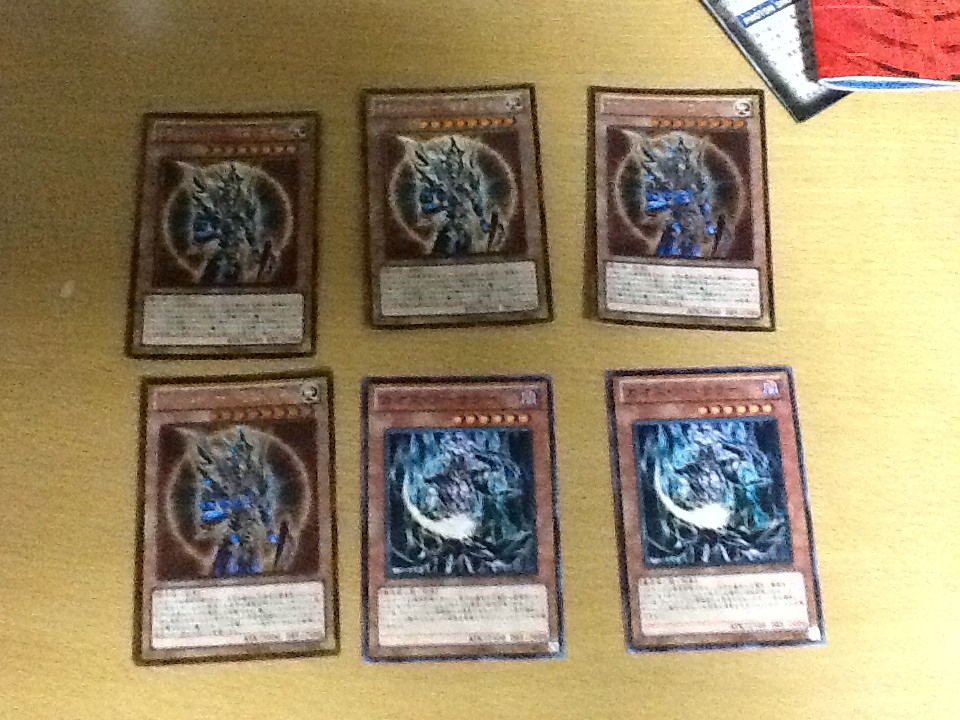The photograph captures six blurred, game-related cards laid out on a light brown or golden cream-colored surface. These cards depict various characters, likely from a role-playing game. The top row consists of three characters with a brown background and a white circle, each featuring an armored figure carrying a large scabbard. The same character appears first on the left in the second row. The last two cards in the second row feature a different character in black armor holding a glowing white sword, placed against a black background with hints of blue. On the right side of the image, there are two manuals - one white with a small blue rectangular box and black text that's illegible, and another red with burgundy lines, showing some white pages with a dark blue section peeking out. The surface appears to be wood grain.